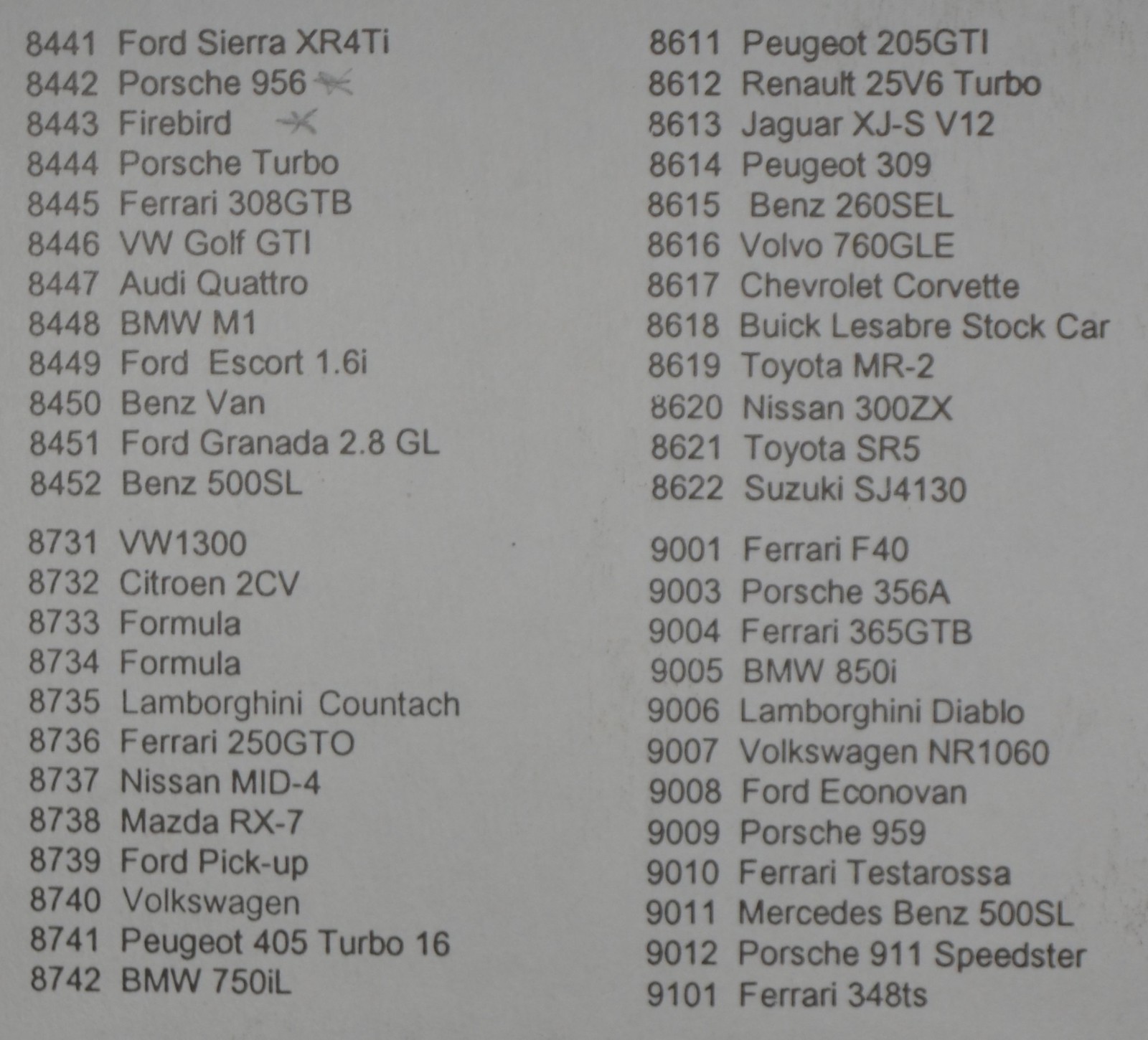The image depicts a slightly grayish sheet of paper featuring a list of various automobile types organized into two main columns, each denoted in regular black font. Each entry begins with a four-digit number followed by the name of the car's brand, model, and type. 

In the upper left corner of the left column, it starts with "8441 Ford Sierra XR4TI." Subsequent entries include a diverse array of vehicles such as "8442 Porsche 956," "8443 Firebird," "8444 Porsche Turbo," and "8445 Ferrari 308 GPB." Lower down in the column, notable listings include "8742 BMW 750 IL."

The right column, which begins with "8611 Peugeot 205 GTI" at the very top, follows a similar structure. Other cars listed here include "8612 Renault 25 V6 Turbo," "8613 Jaguar XJS V12," and a variety of brands such as Buick, Chevrolet, Toyota, Lamborghini, and Ferrari. 

The layout implies a meticulously organized catalog, with each column containing about 30 vehicle entries, providing an extensive overview of multiple car brands and models.